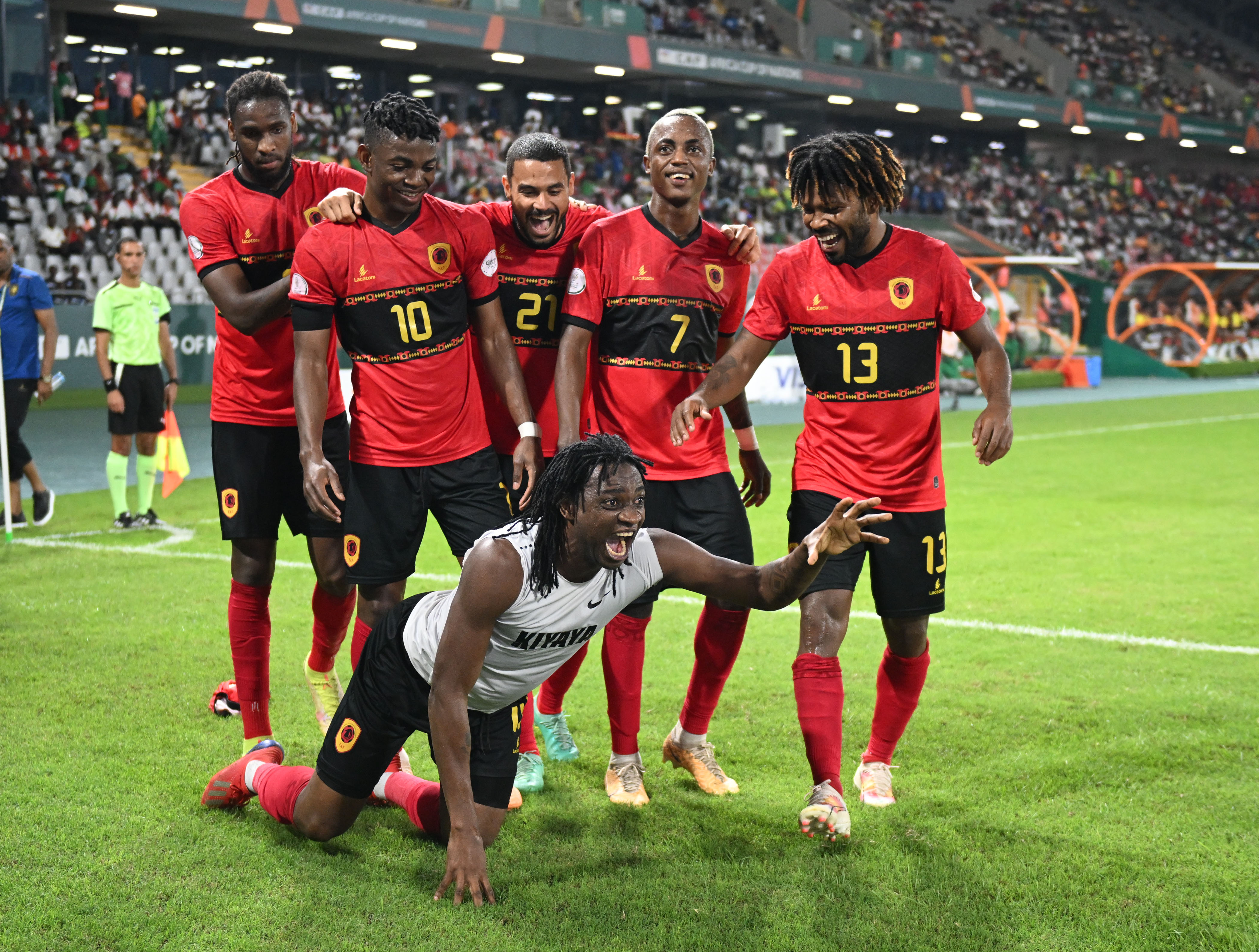A team of six jubilant soccer players is captured mid-celebration on a brightly lit soccer field at night. Five players, standing in red and black jerseys, shorts, and socks, display varying expressions of excitement, while the sixth player, kneeling in red socks, black shorts, and a white jersey, joins in the celebration. Their jerseys are emblazoned with numbers 10, 21, 7, and 13. In the background, a moderately filled stand of spectators watches the scene unfold. A referee, identifiable by his green shirt and referee flags, and a bystander in a blue shirt, partially enter the frame. The vividly green grass contrasts with the night sky, emphasizing the electric atmosphere of the evening match.